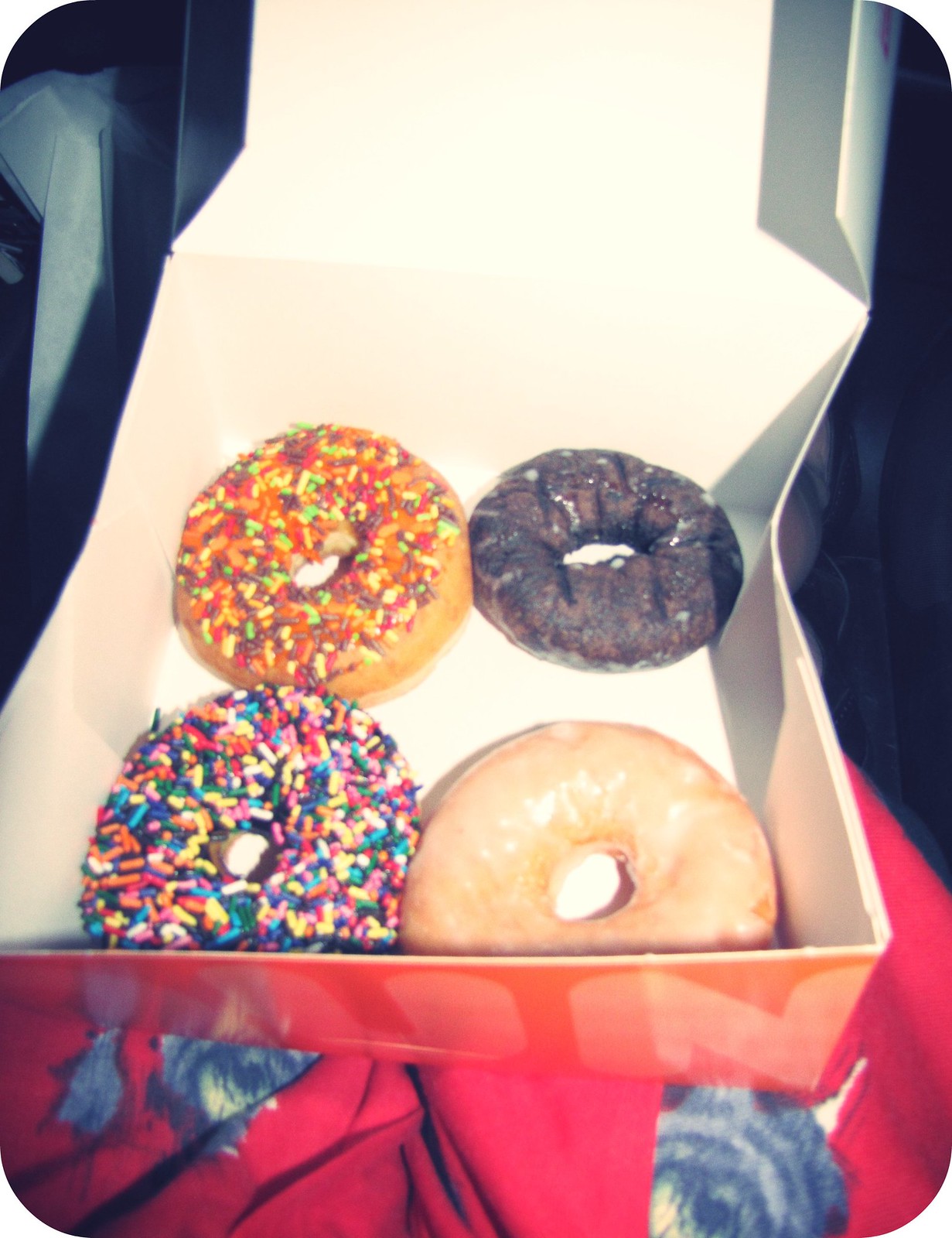The photograph showcases a square doughnut box with an open lid, exposing four round doughnuts with holes in the middle. The box appears to be resting on someone's lap, possibly inside a car, and is positioned over a red felt surface with dog designs. The background is predominantly gray with some textured white and gray material visible on the left side, possibly indicating a seat. Inside the box, the top left doughnut has multicolored sprinkles in yellow, red, and blue, while the top right one is a plain chocolate cake doughnut. The bottom left doughnut also features multicolored sprinkles, though the colors are lighter, including blue and purple. The bottom right doughnut is a simple plain brown doughnut. The vibrant, appetizing doughnuts stand out against the extremely white interior of the slightly bent box.